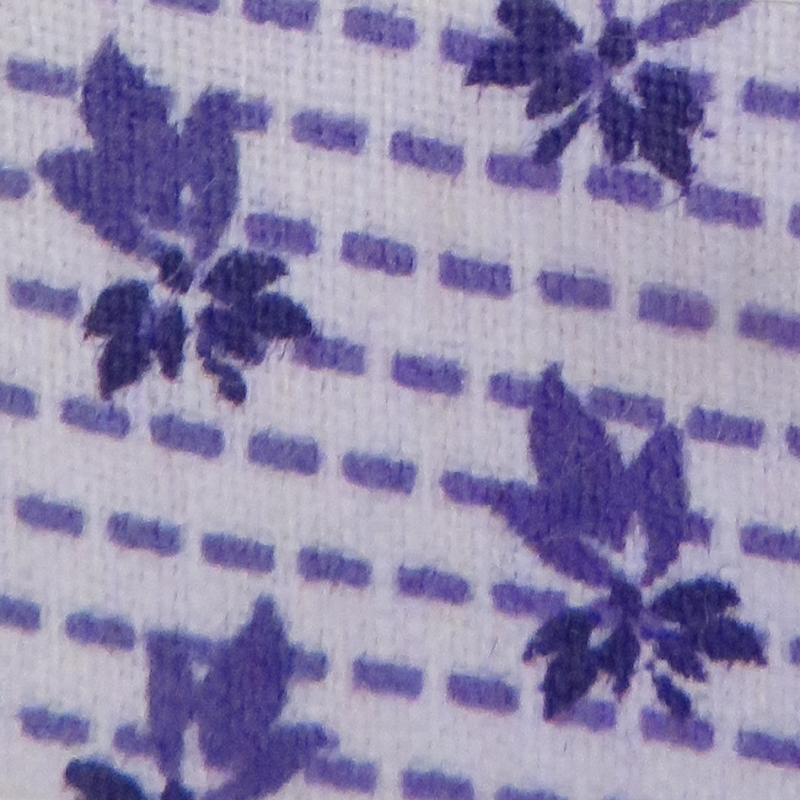This image is an ultra-close-up shot of a white woven fabric, possibly a dishrag or blanket. The fabric features an intricate pattern of several light purple, Morse code-like horizontal dashed lines, approximately seven or eight, arranged in equidistant rows. Interspersed among these dashes are four purple floral or campfire-like designs, with the top part of each motif rendered in a lighter purple and the bottom, showing detailed petals or stacked logs, in a darker purple. The entirety of the design is purple, giving a cohesive yet detailed visual impression. Notably, the flowers are fully visible in the upper left-hand and bottom right-hand corners, while only partial views of the flowers are seen in the upper right-hand and bottom left-hand corners, suggesting a repeating pattern. The entire setup provides a delicate and harmonious interplay of purple hues on a white background, captured in a very detailed macro perspective.